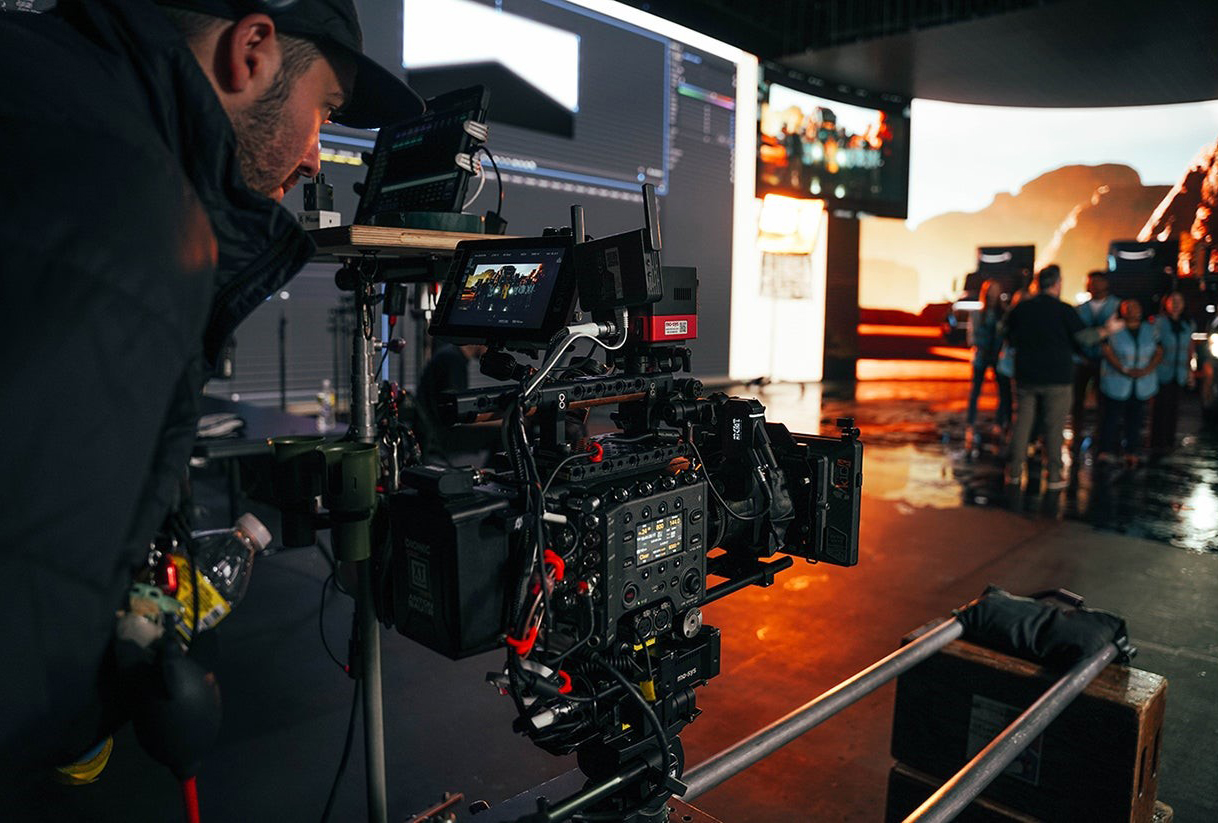In the center of this detailed film studio scene, a man dressed in black stands on the left, his shoulder and head visible. He sports a black baseball cap, showcases brown hair, and has a close-cut beard. The man is intently looking into the viewfinder of an intricately designed camera that is predominantly black with some red accents, featuring a multitude of buttons, dials, and wires. A water bottle peeks out from his jacket pocket, alongside other small items.

Just to the right of the man, the camera captures what appears to be an outdoor Western-themed set with orange mountains and a matching ground. The floor transitions from orange to gray on the right side, where a group of people clad mostly in dark clothing, with one individual in a light blue shirt, stand amidst the set. The background behind them is a mix of gray and black, with a glaring effect caused by artificial sunlight akin to a sunset, illuminating parts of the scene. The upper right corner of the image fades into black, completing this vivid portrayal of a bustling and complex film set.